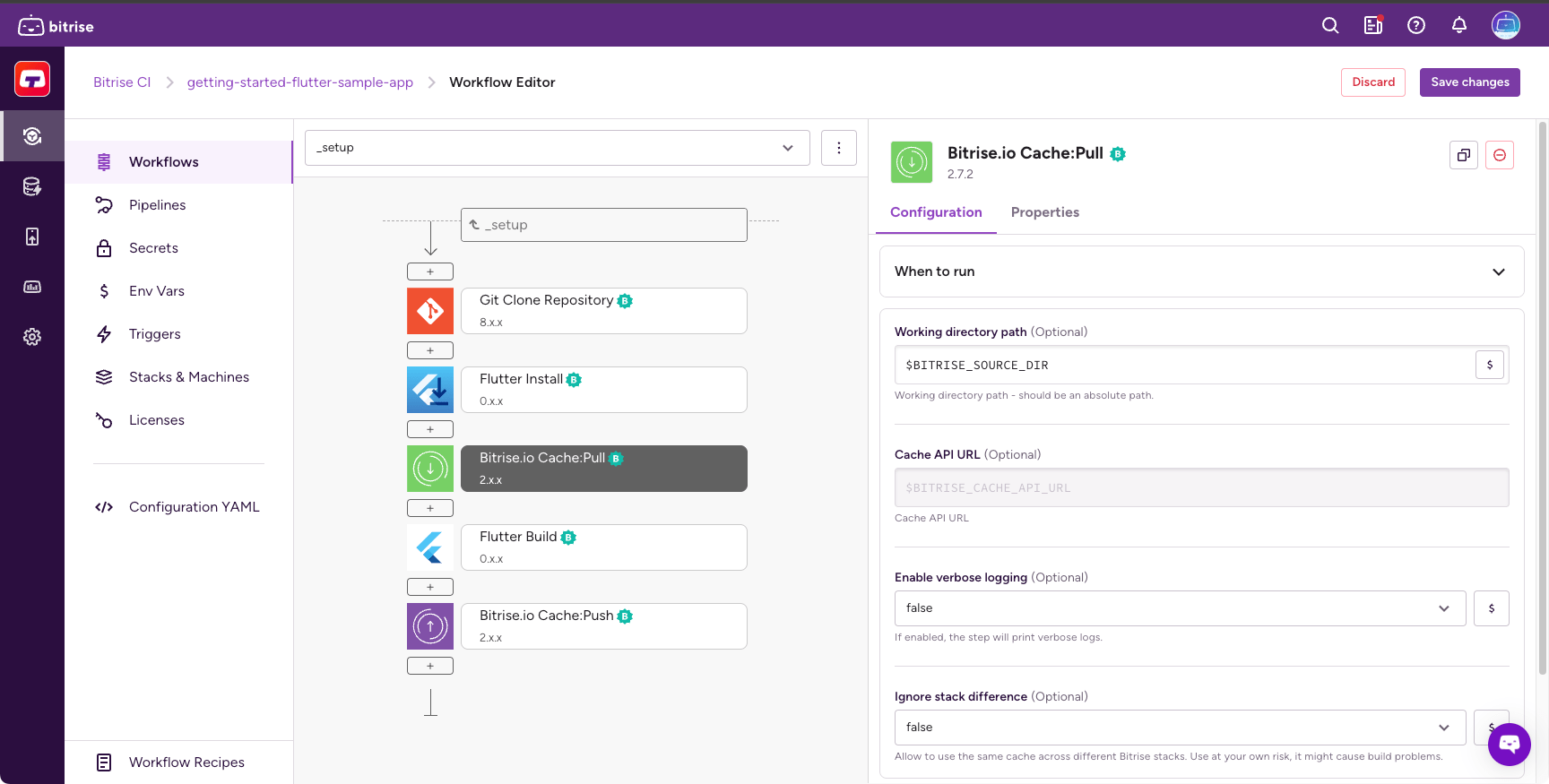This image showcases a user interface with a white background, designed for organizing workflows. At the top of the screen, there is a navigation bar with tabs. The first tab on the left is highlighted in purple and reads "Workflows." Below this tab, there are several buttons labeled "Workflow," "Primary," a plus icon, and three ellipses. In the section under these buttons, several options are presented: "Activate SSH Key," "Git Clone Repository," "Flutter Install," "bitrise.io Cache Pull" (which is currently selected), "Flutter Build," and "bitrise.io Cache Push."

To the right of the "Workflows" tab, there are additional tabs, all in gray: "Code Signing & Files," "Secrets," "Env Vars," "Triggers," "Stacks & Machines," and "bitrise.yml."

The main body of the interface, also set against a white background, contains various settings and editable fields. The first setting is "Working Directory Path," with a corresponding input box showing the value "$BITRISE_SOURCE_DIR." Next is "Cache API URL," with an input box displaying "$BITRISE_CACHE_API_URL." Following this, there is a setting titled "Enable Verbose Logging Required," highlighted in purple, with accompanying text explaining that if enabled, the step will print verbose logs; the current value is "False."

Finally, another setting is "Ignore Stack Difference," which allows the use of the same cache across different Bitrise stacks, though it comes with a warning that it might cause build problems; this option is also set to "False."